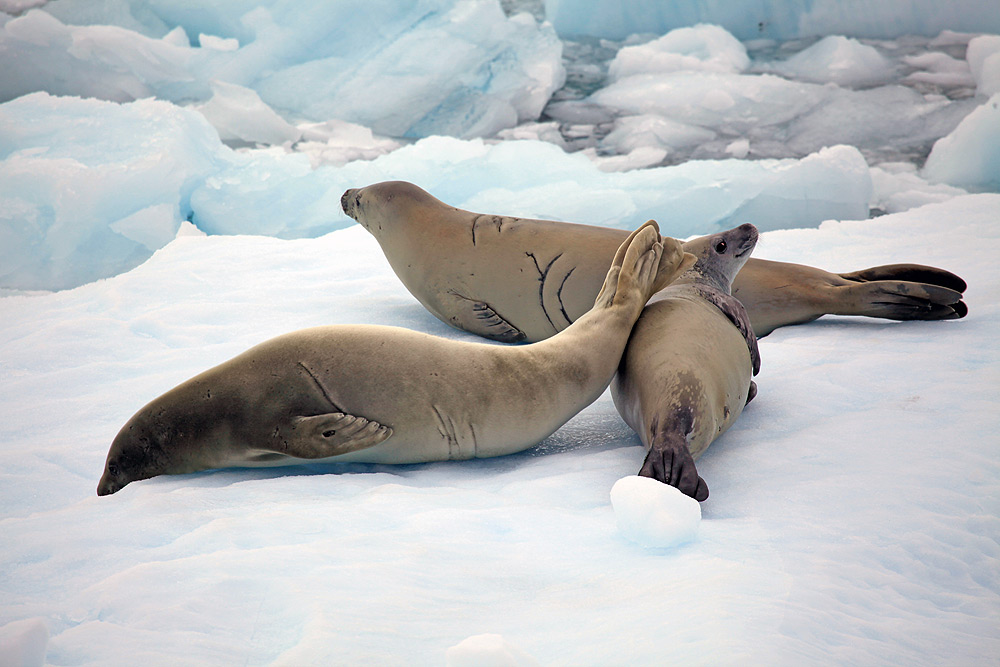This image captures three sea lions resting on a vast expanse of snow-covered ice amidst an oceanic landscape filled with various chunks of ice in shades of white, light blue, and dark gray. The sea lions, positioned at different angles, appear to be content and at ease. The sea lion on the left has its nose pointed downward to the bottom left, its tail resting on the midsection of another sea lion, which is lying with its body facing away from the viewer but looking back towards the camera. The third sea lion, situated in the middle, has its body oriented diagonally left to right, with its head cocked back as if glancing over its shoulder, giving a charming profile shot. Each sea lion's fur transitions from a darker brown at the head to a lighter brown along the body, potentially accentuated by natural scars or markings. The serene backdrop of interspersed ice chunks floating in water enhances the chilly, tranquil atmosphere, devoid of any visible sky or snow beyond the immediate setting.